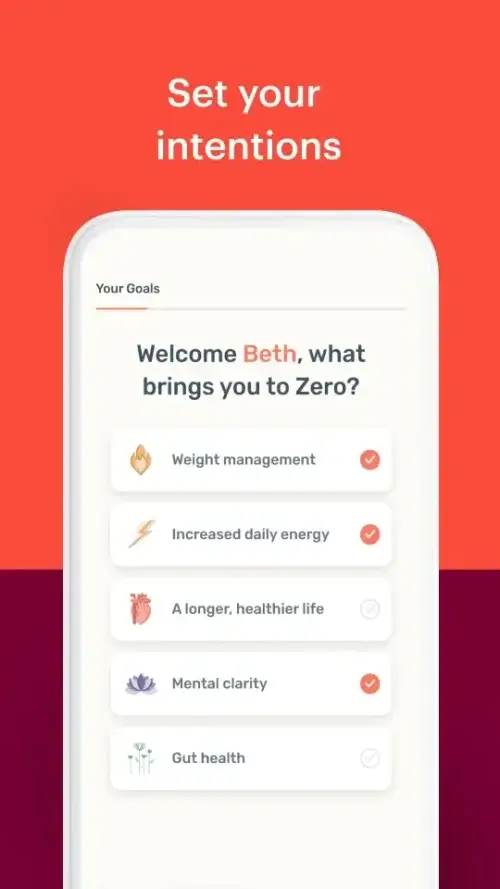In this image, we see a section of a 'Get Started' page for weight loss and wellness. The page features text prompting users to "Set your intentions and your goals." 

At the top, there is a personalized greeting, "Welcome Beth," followed by the question, "What brings you to Zero?" Underneath, a list of health and wellness goals is displayed with checkboxes for tracking progress:

- Weight management (checked)
- Increased daily energy (checked)
- A longer, healthier life (not checked)
- Mental clarity (checked)
- God's health (not checked)

The checkboxes allow users to mark their specific goals for clarity and motivation. The interface design uses shades of orange and red against a white background, providing a vibrant and clean visual appeal.